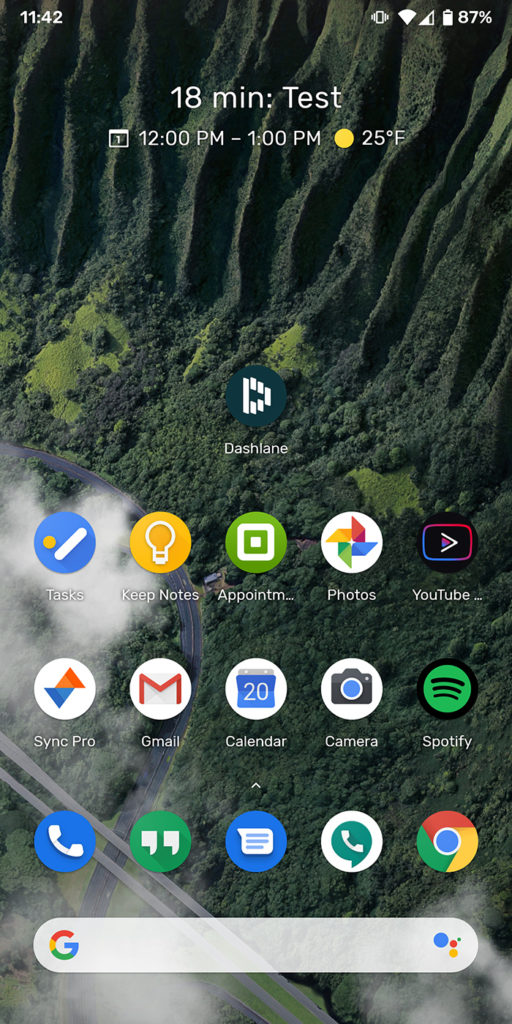The image showcases a phone screen displaying a notification over a picturesque background. The orientation is portrait, roughly twice as tall as it is wide, fitting typical smartphone dimensions. The background image is a stunning high overlook of a mountainous area filled with dense trees, winding roads, and a layer of clouds and fog settling in the valleys below, creating a serene and picturesque scene.

At the top of the screen, in white text, the time is displayed as 11:42, situated either in the upper right or left corner. To the upper right, various status icons are visible: a vibrate mode icon, a fully filled Wi-Fi meter, a network connection gauge at approximately 75%, and a battery indicator showing 87% with a vertical battery icon.

The header of the phone screen reads "18 minute test," followed by a scheduled event from 12 p.m. to 1 p.m., denoted by a sun icon and a temperature reading of 25 degrees Fahrenheit. Below this, a single icon for "Dashlane" is prominently displayed above a grid layout.

The main grid consists of five columns of three icons each, displaying apps such as Tasks, Keep Notes, Appointments, Photos, YouTube, Sync Pro, Gmail, Calendar, Camera, and Spotify. At the very bottom of the screen, generic icons provide quick access to Phone, Messaging, Texting, Phone Calls, and Google Chrome. Additionally, there's a gray Google search bar with a "G" icon on the extreme bottom.